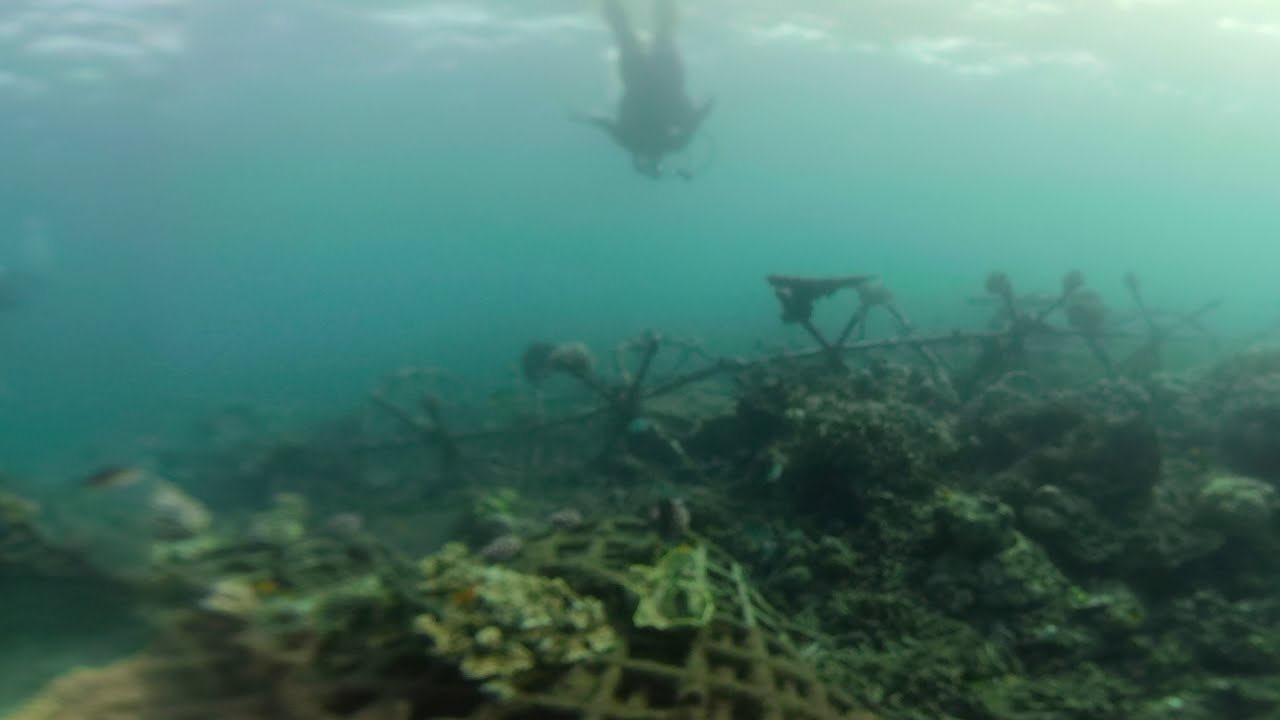An underwater scene captures a scuba diver descending through murky, cloudy blue-green water typical of the ocean. The diver, equipped with full scuba gear, swims towards a debris-strewn ocean floor that is partially illuminated by diffused sunlight from above. The seabed features an array of rocky formations and large patches of algae, interspersed with remnants of man-made structures. Among the wreckage, one can discern a long tree branch, fragments of machinery, and a submerged metal frame, all encrusted with rust and algae, suggesting an old shipwreck or abandoned underwater site. The backdrop is dreary and blurry, adding to the mysterious and eerie ambiance of the scene.